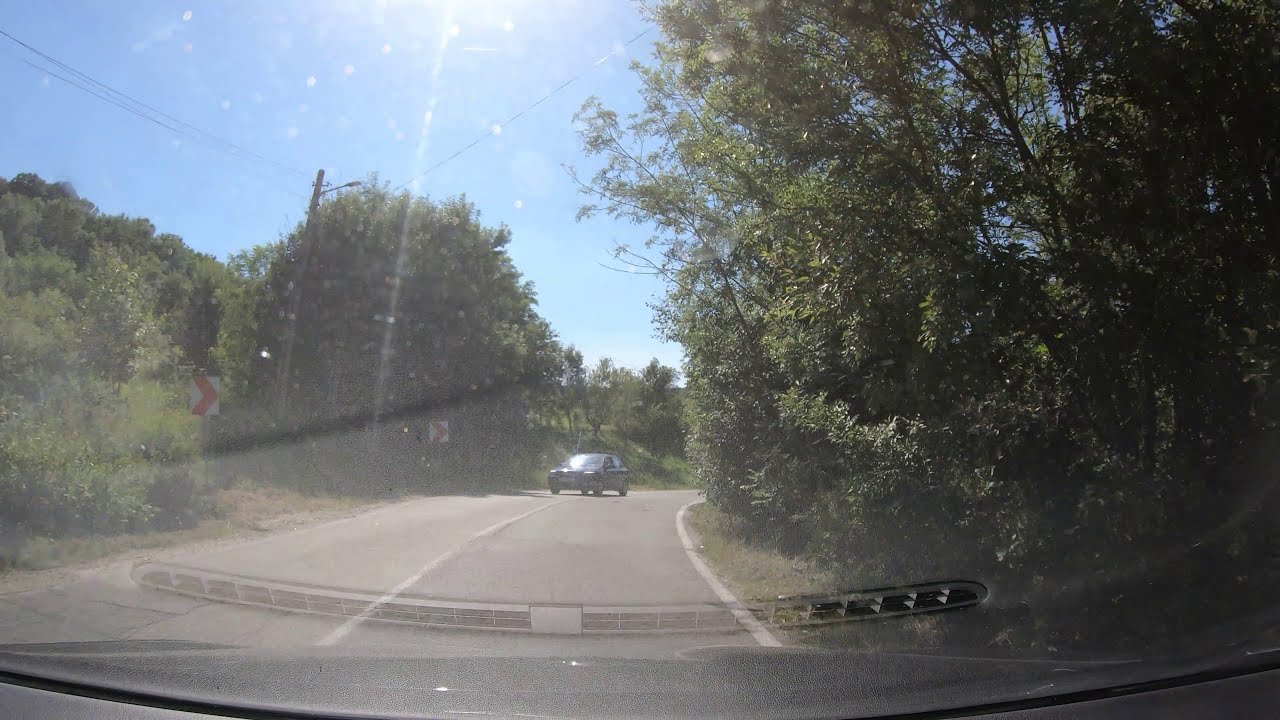A photograph taken from the dashboard of a car reveals a two-lane country road curving to the right. Trees and dense bushes flank the road, their branches overhanging slightly. The reflection of the car’s air vents is visible at the bottom edge of the windshield. Ahead, a dark-colored sedan is emerging from around the bend, about 20 feet away. Street signs on the left side mark the road's curve, while a streetlight stands nearby. A cloudless, bright blue sky completes the serene rural scene.